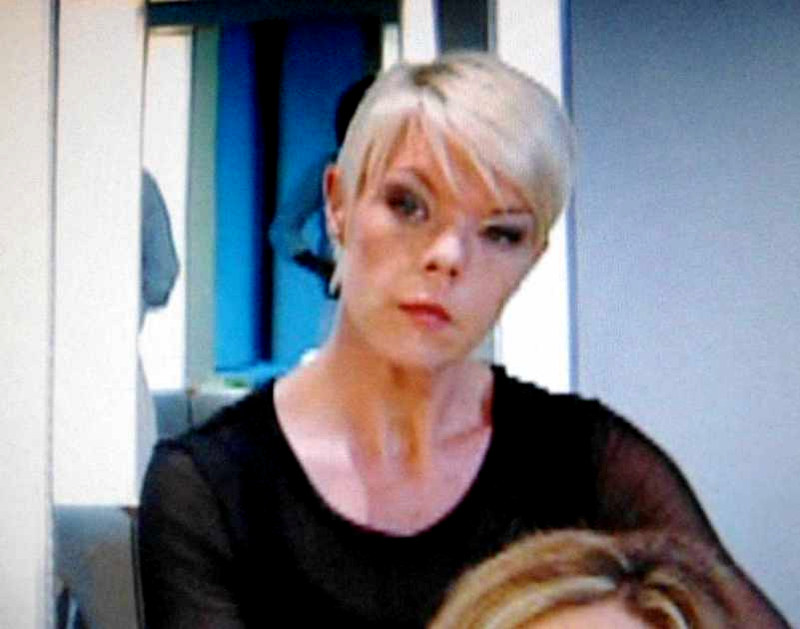The image captures a young celebrity woman, known for her appearances on HGTV where she renovates beauty salons, sitting behind another individual. The focus is sharp on her, revealing her pointed and drawn face with very arched eyebrows enhanced by heavy eye makeup. She sports a very short, white blonde pixie cut and is clad in a thin, long-sleeved black shirt. Just in front of her, the top of another person's head is visible, featuring blonde hair with darker blonde streaks, likely suggesting she might be a hairdresser at work. The background reveals a mirror flanked by vertically-hung LED lights, with the surrounding people and white walls appearing blurry, further emphasizing the central figure.